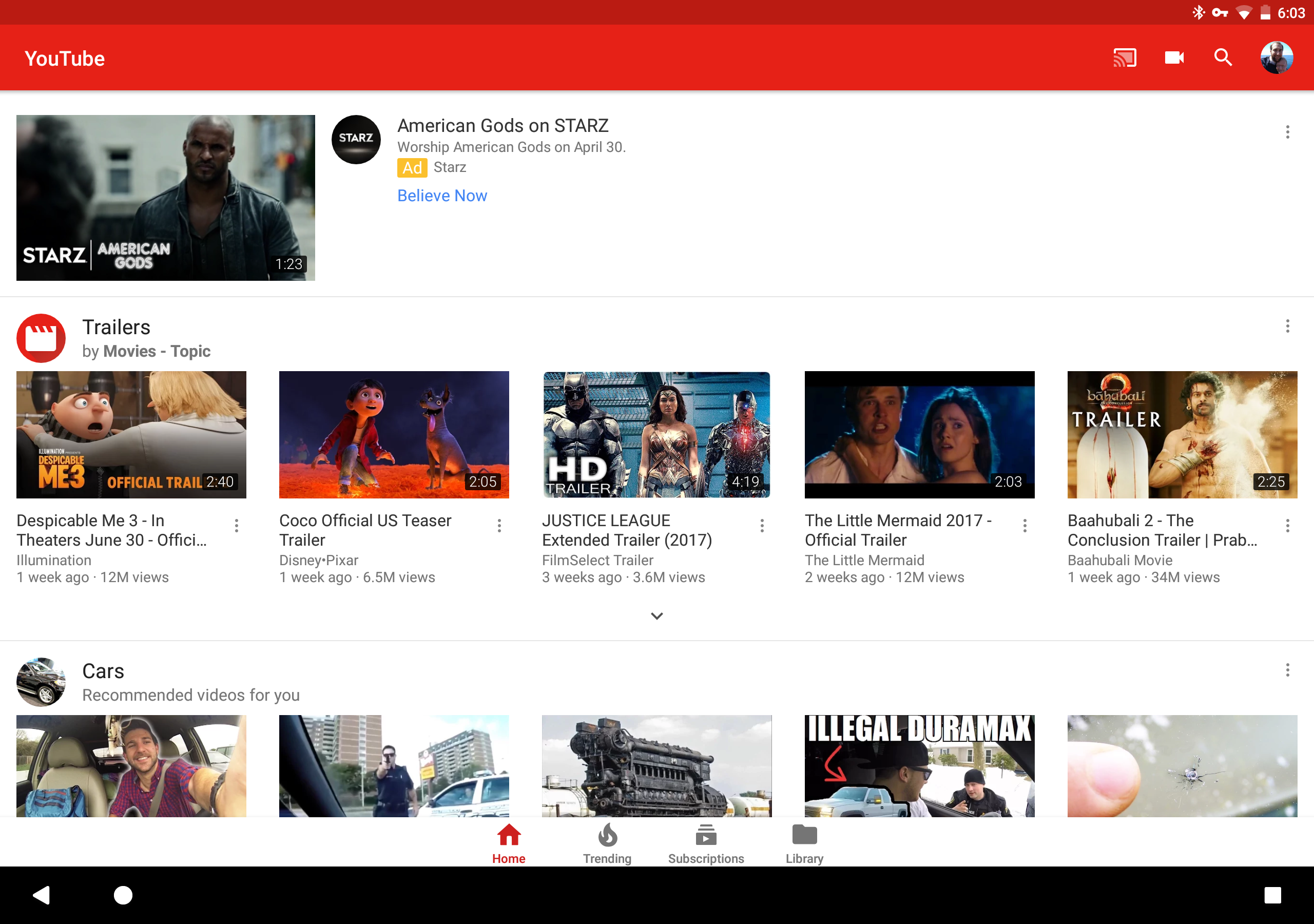The image features a web page with a prominent red border at the top. The top-left corner displays the YouTube logo, while the top-right corner is populated with various icons including one for full-screen mode, a camera, a magnifying glass, a profile picture, and the current time among other typical interface symbols. 

Below this header, the page transitions to a white background. On the top left, there is a still from a movie with text indicating "American Gods" on Starz, trailing the phrase “Worship American Gods.” It notes the duration of 1 minute and 23 seconds with the upcoming airing date specified as April 30.

Beneath this section is a carousel of video thumbnails and titles running horizontally from left to right. The first thumbnail promotes "Despicable Me 3 in Theaters June 30" by Illumination, uploaded one week ago with 1.2 million views. Next to it, there's a thumbnail for "Coco Official U.S. Teaser Trailer" by Disney Pixar, also uploaded one week ago, but with 6.5 million views. The last visible thumbnail advertises the "Justice League Extended Trailer 2017."